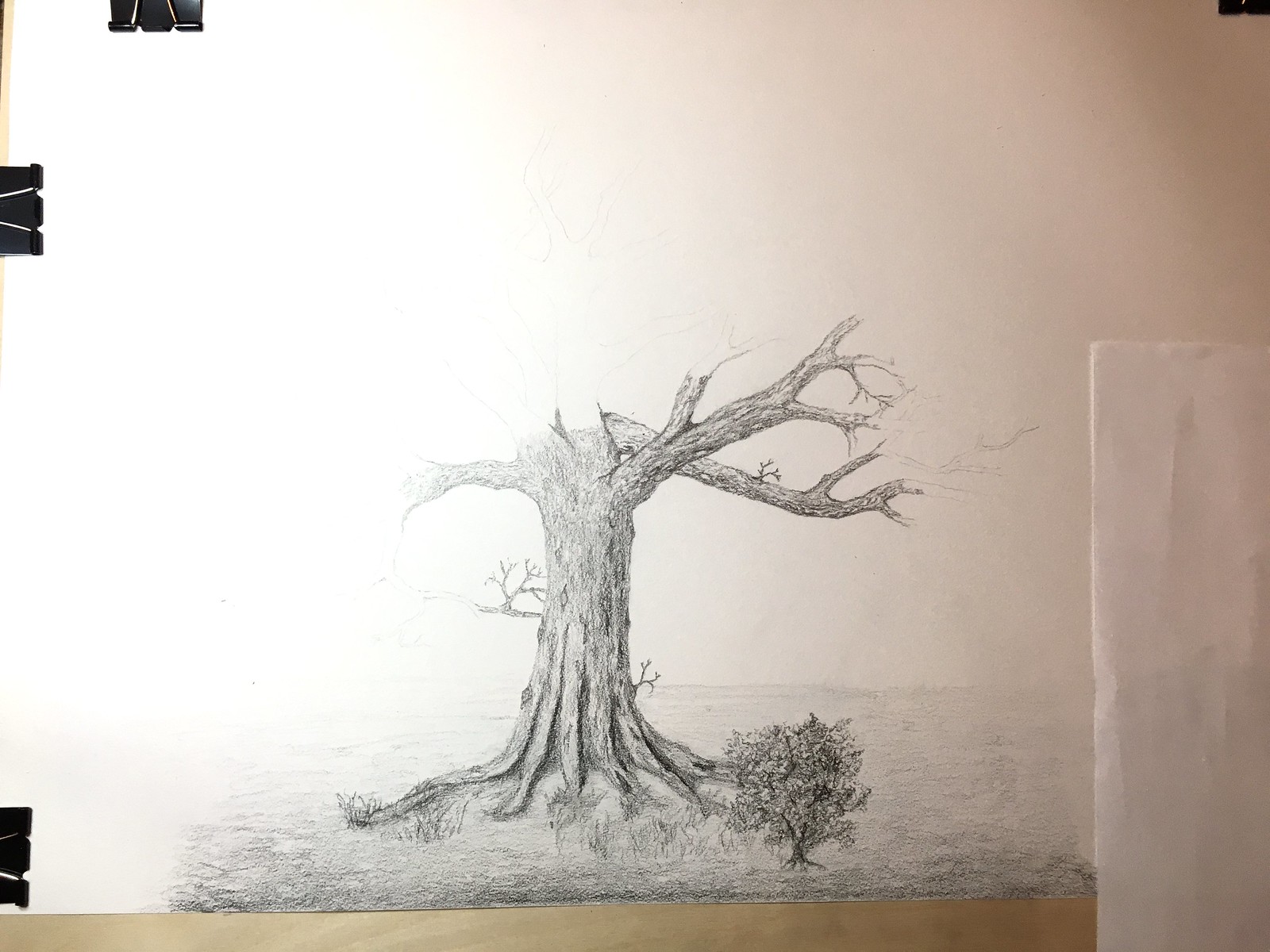A detailed pencil sketch illustrates a serene field dominated by a prominent dead tree. The tree trunk is meticulously shaded and completed, showcasing intricate textures and shadows. Surrounding the base, tufts of grass intertwine with the trunk, enhancing the natural feel of the scene. However, the tree’s branches remain in preliminary phases, with faint outlines suggesting the sprawling structure still in progress. 

On the bottom right-hand side of the trunk, a small, fully realized shrub stands out, replete with detailed leaves, contrasting with the unfinished branches. The drawing itself is secured with black paper clips at the edges, ensuring it remains steady and undisturbed as the artist continues their work.